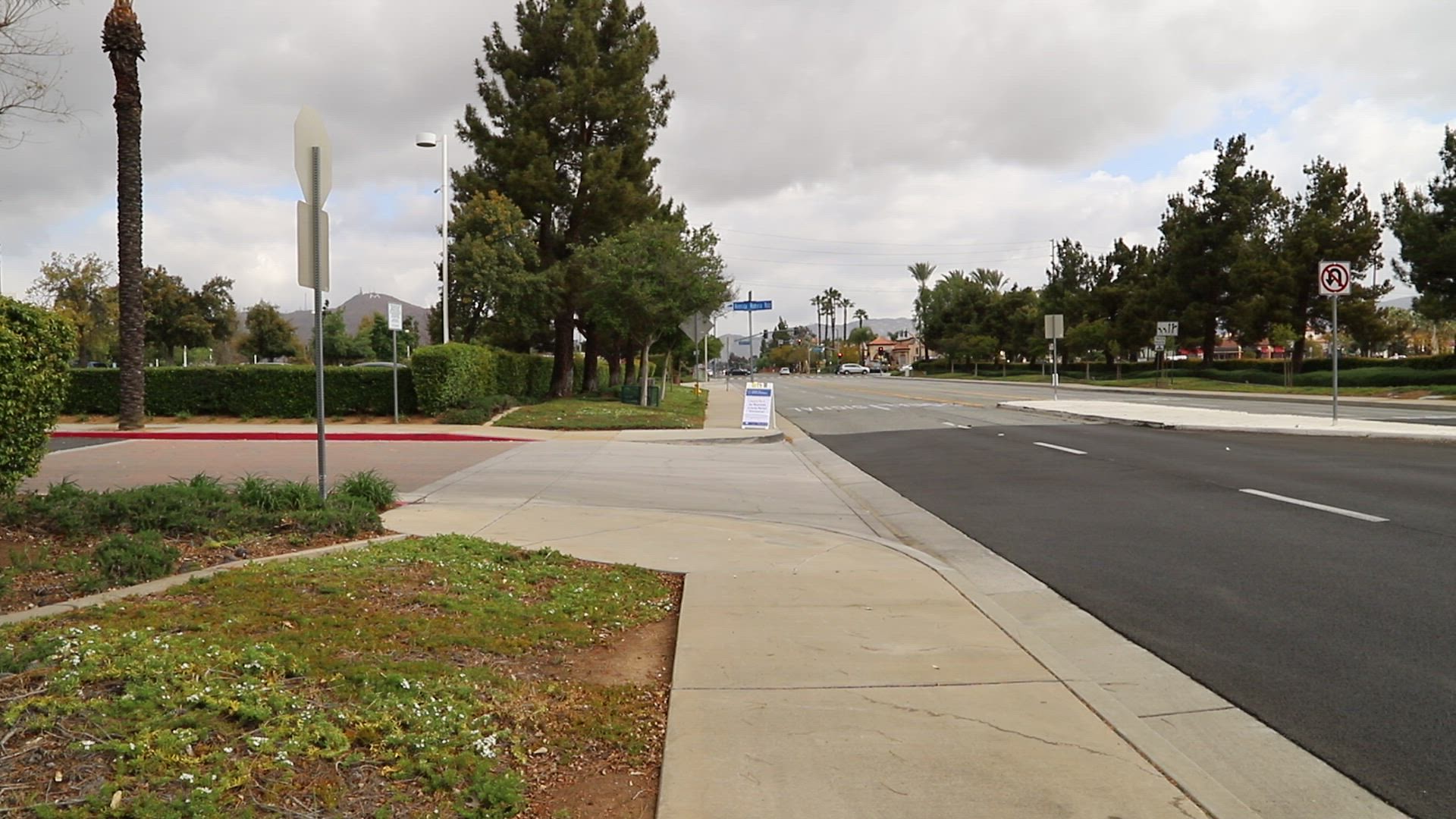The photograph depicts a street scene with minimal vehicular traffic, emphasizing a contrast between the dark, newly-repaired asphalt and a lighter-colored section of the road. The perspective is from a sidewalk, extending both straight down the street and to the left, where an unkempt area filled with ground and weeds contrasts with a more cultivated space further left. 

A tall palm tree stands prominently across what might be a side street or entryway, forming a T-intersection. The intersection features a traffic median that restricts turns and prevents U-turns, suggesting it’s primarily an entrance point. Across this median, the opposite lanes of the highway are visible, lined with trees and accompanied by a grassy area and a sidewalk along Mass Street 2.

In the distance, various street signs, palm trees, other types of trees, and buildings hint at a suburban environment. The sky above is mostly cloudy, with occasional patches of blue peeking through, adding to the expansive and open feel of the suburban landscape.